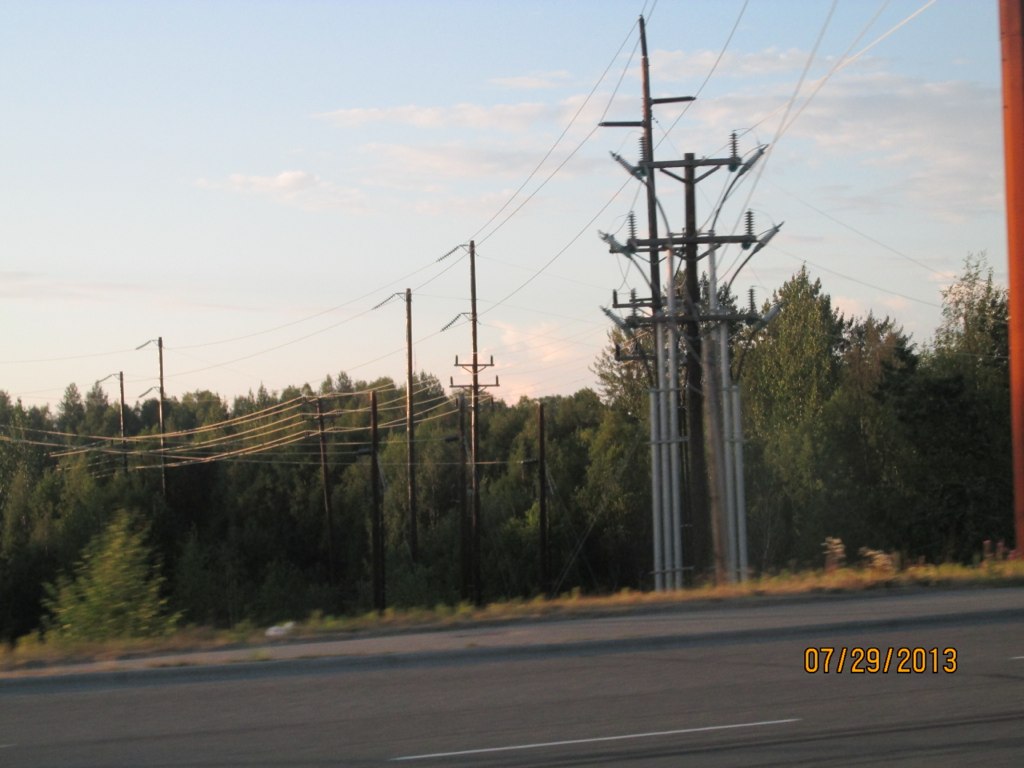The photograph, taken on 07/29/2013 as noted in the yellow text in the bottom right corner, captures a roadside scene with a gray road prominently featuring a singular white lane line. Running parallel to the road is a sidewalk, beyond which lies a field ditch out of view. Dominating the middle ground are numerous telephone poles, varying in thickness and color—some are tall and dark brown, others slender and silver—with an intricate network of wires connecting them. Flanking these poles is a dense line of green-leaved trees suggesting a deep forest in the background. Above this arboreal density, the bright blue sky is adorned with drifting gray clouds, suggesting it is daytime with clear lighting. The scene, likely captured from a moving vehicle, is complemented by brown grass patches along the roadside, contributing to the overall impression of a tranquil yet unglamorous rural landscape.